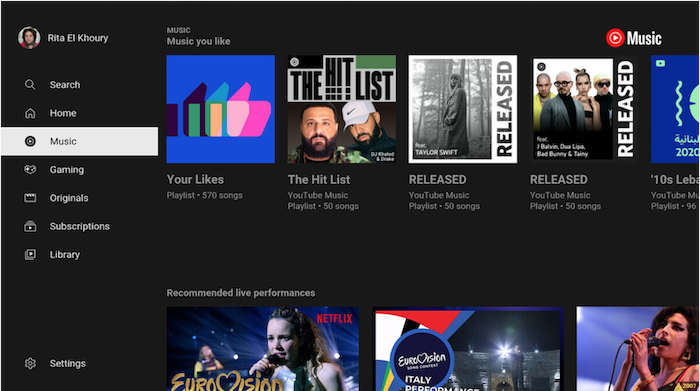The image displays the homepage of the YouTube Music app, featuring a two-column layout with a menu on the left and content on the right. At the top left corner of the menu, there is an avatar featuring a picture of a woman, labeled with the name "Rita Al-Khoury," indicating the account holder. The menu items, each accompanied by a corresponding line art icon, include options such as Search, Home, Music, Gaming, Originals, Subscriptions, Libraries, and Settings at the very bottom.

On the right side of the interface, there are several album or playlist covers displayed in a consistent ratio, labeled under "Music" with a subtitle "Music You'd Like." Highlighted playlists include:
- "Your Likes" – Playlist with 570 songs.
- "The Hit List" – YouTube Music playlist with 50 songs.
- "Released" – Another YouTube Music playlist with 50 songs.
- "Lebanese Music" – YouTube Music playlist containing 96 songs, partially cut off.

Below these playlists, there is a section titled "Recommended Live Performances," showcasing thumbnails of various videos. At the very bottom right corner of the page, there's a thumbnail featuring the singer Amy Winehouse. The content is partially cut off at this point, leaving some details obscured.